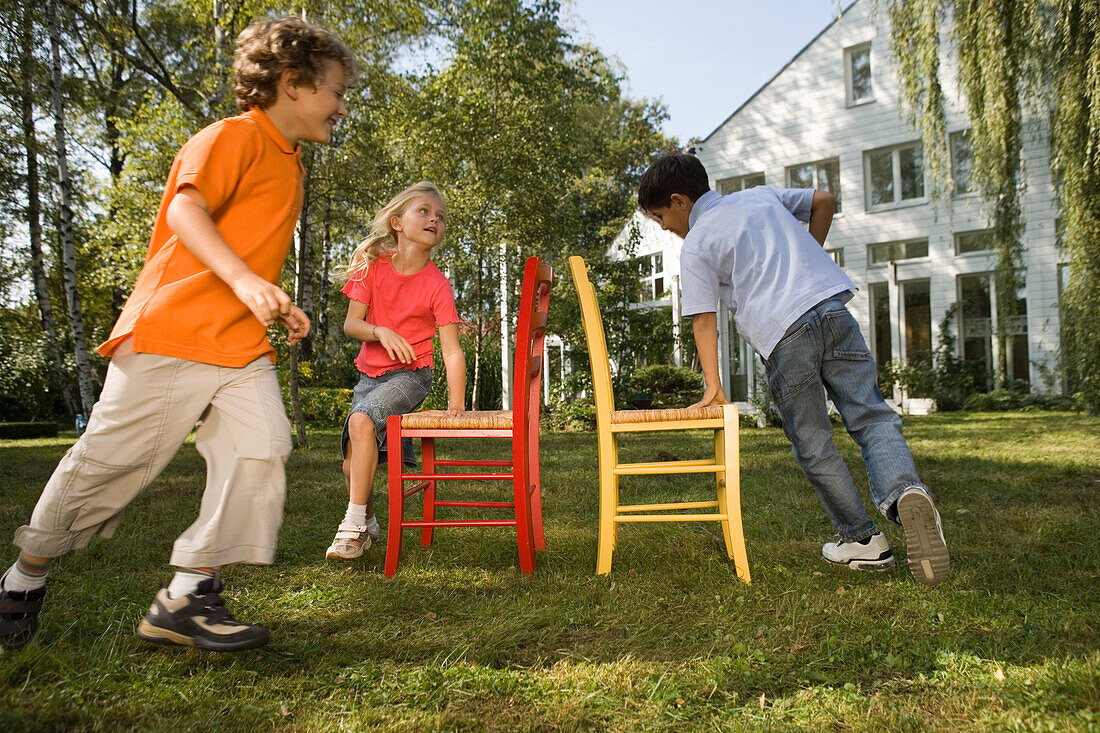In a picturesque grassy yard, three small children, two boys and a girl, are captured in an energetic game of musical chairs. They are running clockwise around two back-to-back chairs—one red on the left and one yellow on the right. The boy on the far right, wearing a blue polo shirt, jeans, and white shoes, has dark hair and slightly darker skin. His left hand rests on the chair as he runs. In the middle, the young girl, with blonde hair and lighter skin, sports a red shirt and denim shorts with white shoes, also touching the chair with her left hand. Closest to the viewer, the third child, a boy with light brown hair and slightly darker skin, races around in an orange polo shirt and khaki cargo shorts.

Surrounding the children, the green yard is bordered by lush trees. To the left, there is a dense cluster of tall trees, while on the right, the delicate leaves of a weeping willow dangle down. The backdrop features a modern-style white house, characterized by its three stories and numerous large windows. Notably, the top floor showcases long, floor-to-ceiling windows, adding an elegant touch to the scene, while the second floor has a row of windows and a single window near the angled roof. The overall setting captures the joys of outdoor play on a sunny day.